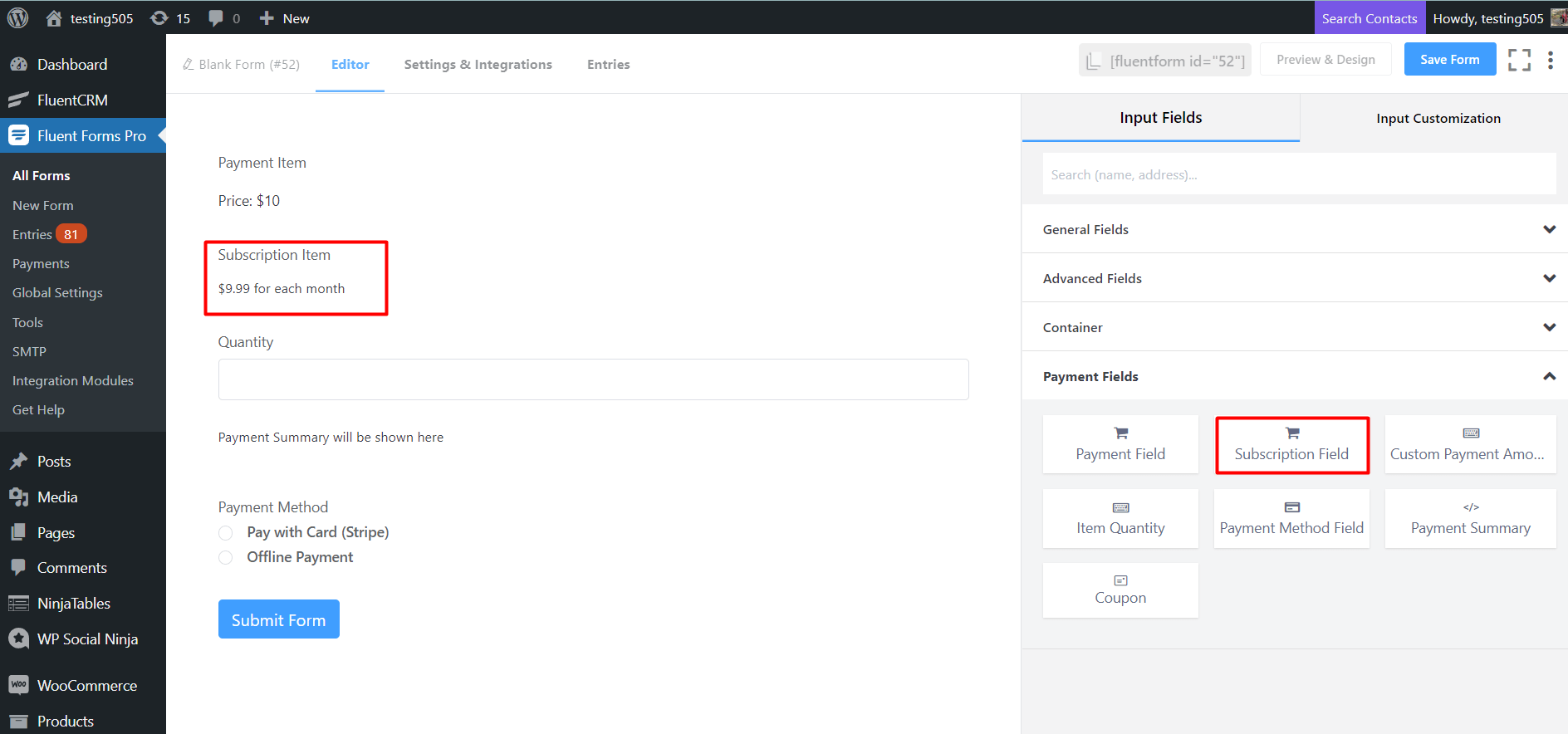Here's a detailed and cleaned-up caption for the given image:

---

The image is a screenshot taken from a WordPress site showcasing various admin functionalities, primarily focusing on a form editor interface. At the top of the image, there are search functionalities and a "Howdy, testing 505" greeting message. 

On the left side, a vertical dashboard menu is visible, featuring options such as FluentCRM, Fluent Forms Pro, All Forms, New Form Entries (81), Payments, Global Settings, Tools, SMTP Integration Modules, Get Help, Posts, Media, Pages, Comments, Ninja Tables, WP Social Ninja, WooCommerce, and Products. 

Highlighted within this menu is "Form Number 52," showing options like Editor, Settings and Integrations, Entries, Fluent Form ID equals 52, Preview and Design, Save Form. Below these, specific form fields include "Payment Item" priced at $10, and a "Subscription Item" costing $9.99 per month. There are fields for quantity input and a blank space for additional data across the form, followed by a summary area labelled "Payment Summary will be shown here" and payment methods options, including "Pay with Card," "Stripe," and "Offline Payment." The form concludes with two radio buttons for payment method selection and a "Submit Form" button.

On the right side, a detailed section named "Input Fields and Input Customization" is presented, with the "Input Fields" tab currently active and highlighted with a blue underline. Within this tab, there are search fields for Name and Address alongside a searchable box, and options to access "General Fields" and "Advanced Fields," both expandable. Additional tabs like "Container" and "Payment Fields" can be clicked to reveal further options. The "Payment Fields" tab is expanded, showcasing individual boxes for "Payment Field," "Subscription Field" (highlighted in red), "Custom Payment Amount," "Item Quantity," "Payment Method Field," "Payment Summary," and "Coupon." Each box is marked with distinct icons resembling shopping carts or card images.

---

This detailed caption provides a clear and comprehensive description of the image's contents, making it accessible and understandable.